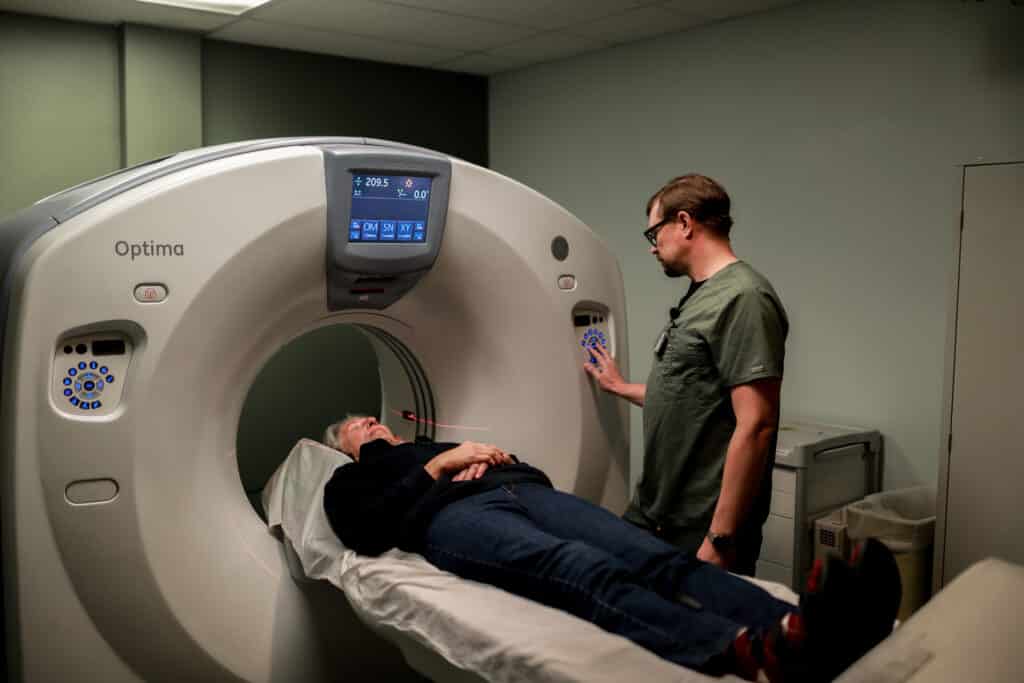In this detailed landscape photograph, an elderly Caucasian man with white hair is seen lying on a white sheet-covered table, preparing to enter a light beige MRI machine labeled "Optima." He is dressed in a black long-sleeve shirt and black pants, with his hands folded over his chest. His head rests on a white-cushioned pillow. Adjacent to him, a Caucasian male technician in his 40s, distinguishable by his brown hair, glasses, and green short-sleeve scrub top, operates the machine with his right hand, which has a watch on the left wrist. The MRI machine features a variety of circular blue buttons and a dark gray frame surrounding a navy blue touchscreen. The background reveals a light-colored ceiling and walls, a section of greenish light from fluorescent bulbs, and glimpses of a door and a trash can. The overall focus of this image remains on the patient readying for his scan and the technician diligently working the controls.